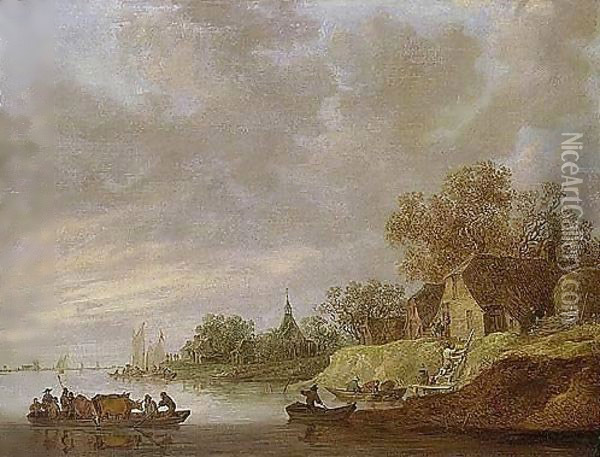This is a grainy image of a painting depicting an outdoor riverside scene. In the foreground, a small, loaded canoe with several people and a couple of cows is stationed at the bottom right corner, near a steep cliffside shore. Adjacent to it, in the center bottom of the image, a lone man paddles another canoe close to the shore. The cliff, brown on its sides with a green top, supports a house with a noticeably sloped brown roof and green front wall. Behind the house, tall trees laden with green leaves rise up. In the background, more up the river to the center and right, boats with sails can be seen in the distance, and the tip of a church steeple protrudes into the sky. The sky is filled with a dramatic mix of dark gray and dark yellow clouds. Vertical text on the right side reads "NiceArtGallery.com," contributing an additional layer of context to the image. The entire scene is captured in a variety of colors including light green, gray, tan, brown, dark brown, a bit of black, and off-white. The portrayal suggests a calm yet lively riverside moment, with boats arriving and nearby homes blending into the natural environment.